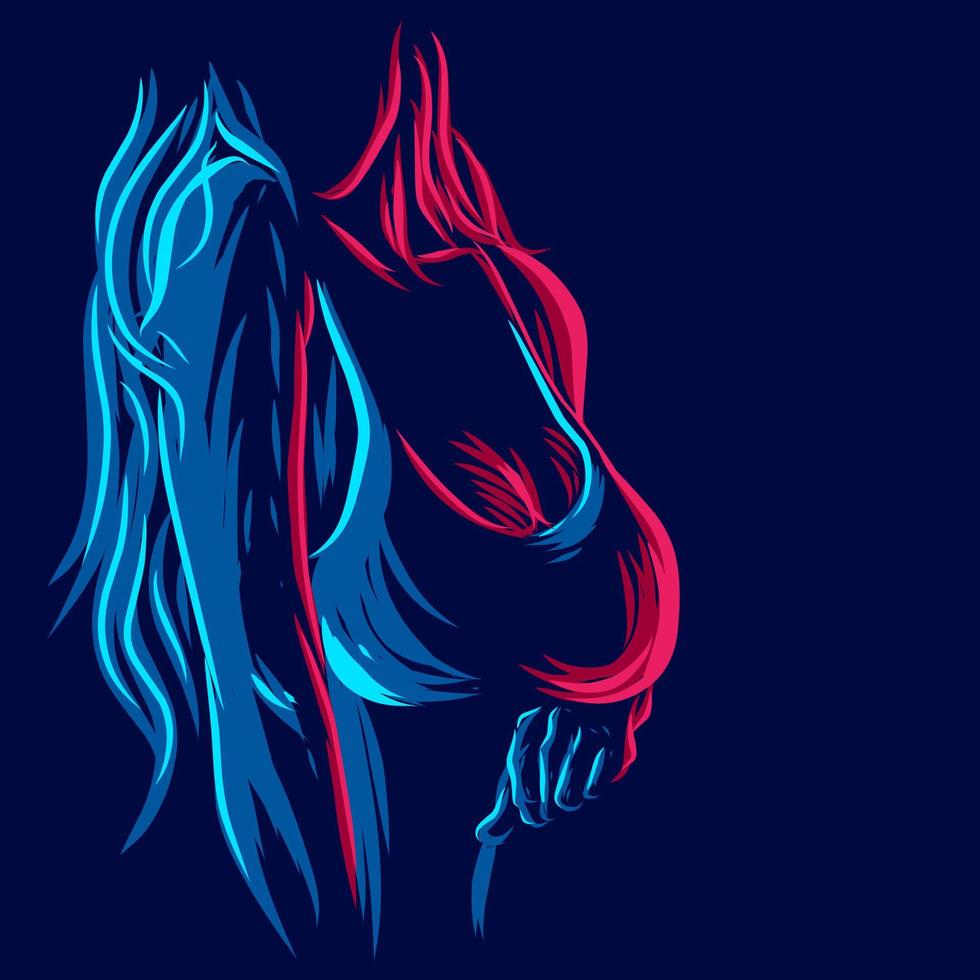The artwork, which appears to be a painting or graphic, is set against a dark blue, almost black background and is arranged in a square format. Dominating the center, slightly towards the left, is the silhouette of a woman with intricate, long, flowing hair. Her hair displays a striking contrast with its vibrant colors; one side is predominantly a pink to maroonish hue while the other side transitions from light blue to a medium blue. Her head tilts slightly towards the viewer, with the hair cascading down her shoulders in layers. Despite the large and prominent breasts, which would typically lend a sense of sexiness, the way they are depicted gives a somewhat hairy appearance, adding an unsettling twist.

The woman's left hand, which is highlighted in blue, extends outward and seems to merge with the contoured outline of her body, creating a surreal effect. There is notable attention to the hair's texture and flow, with a single red stripe accentuating the blue side. In the pinkish hair, a cradle-like shape forms around the hand, suggesting that something could be nestled within. The overall visual gives a sense of allure mixed with ambiguity, hinting at the possibility of a strip club sign while retaining an artistic, almost abstract quality.